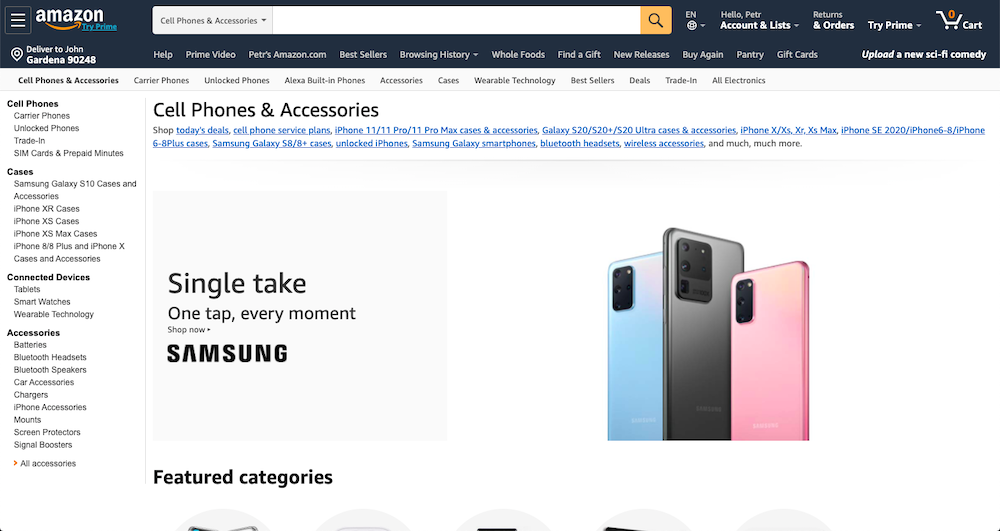This screenshot captures the top section of a website viewed in a browser, featuring a dark blue header. On the far left of the header, there is a white hamburger menu icon, outlined with a thin medium gray square. Next to it, the word "amazon" is displayed in all lowercase white text, with an orange concave arrow beneath that starts at the bottom left of the "M" and ends at the bottom of the "Z," partially obscuring the latter. 

To the right of the logo, blue underlined text reads "tri-prime." Moving further right, after a small gap, there is a search bar. The search bar's left side contains a light gray rectangle with dark gray text that reads "cell phones and accessories," accompanied by a dark gray downward-pointing arrow. A thin, medium gray vertical line separates this section from the adjacent white text box, which is empty. Attached to the right side of the text box is an orange square with a dark blue magnifying glass icon.

Continuing to the right, there's the text "EN" in white, and below it, a white globe icon with a grid design, flanked by a light gray downward-pointing arrow. The remaining space is divided into three columns of text. The first two columns feature a line of smaller light gray text above a line of larger white text. The first column reads "Hello Peter," followed by "accounts and lists" and a white downward-pointing arrow. The second column reads "returns" in light gray and "orders" in white. The third column only contains the larger white text "tri-prime" with a light gray arrow pointing down beside it.